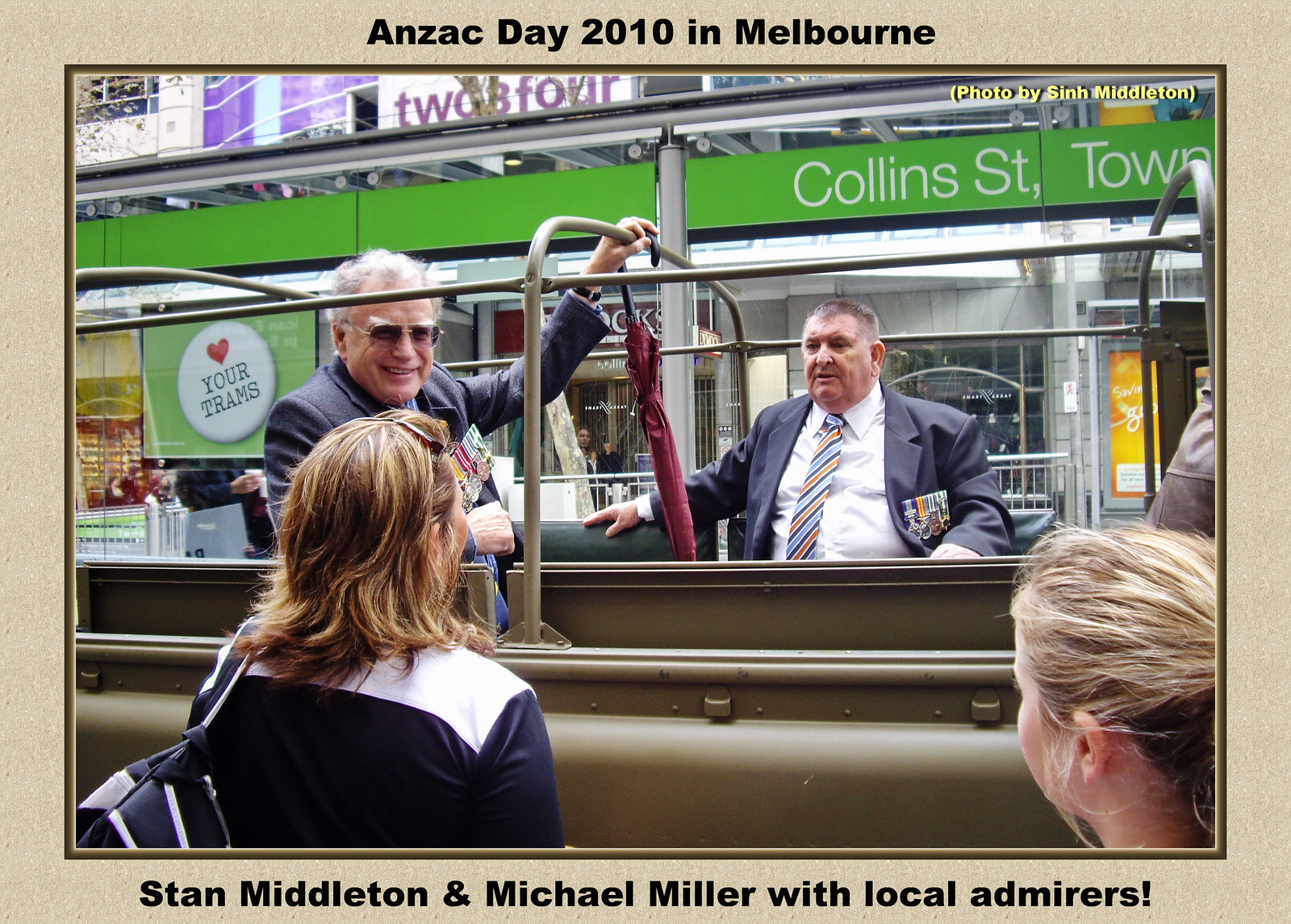The photograph captures a vivid scene from Anzac Day 2010 in Melbourne, as denoted by the text on the tan-colored top border. Encased in a tan and thin brown frame, the bottom border further identifies "Stan Middleton and Michael Miller with local admirers" in black text. The central image showcases two elderly men seated in the back of an open-air military truck, notably painted brown, likely part of a parade. 

The man on the left, Stan Middleton, sports fuzzy white hair, prominent white eyebrows, dark sunglasses, and a blue business coat adorned with a row of medals on his left chest. He holds a red umbrella in his right hand. Adjacent to him is Michael Miller, a heavier-set man with short dark hair, dressed in a suit with a blue and orange striped tie over a white shirt, also decorated with an array of medals.

In the foreground, two women stand with their backs to the camera, conversing with the gentlemen. The woman on the left, dressed in a blue jacket with a white overlay and carrying a blue and white shoulder bag, has her hair tied back. Next to her, only the back of a second fair-haired woman's head is visible.

The backdrop hints at a bustling city street with shopfronts and tall buildings. A prominent green banner reads "Collins Street," and a white circular sign featuring a red heart advocates for "Heart your trams." In the top right corner, faint yellow text credits the photograph to Sinh Middleton. The scene is rich with details, capturing a moment of camaraderie and historic remembrance.